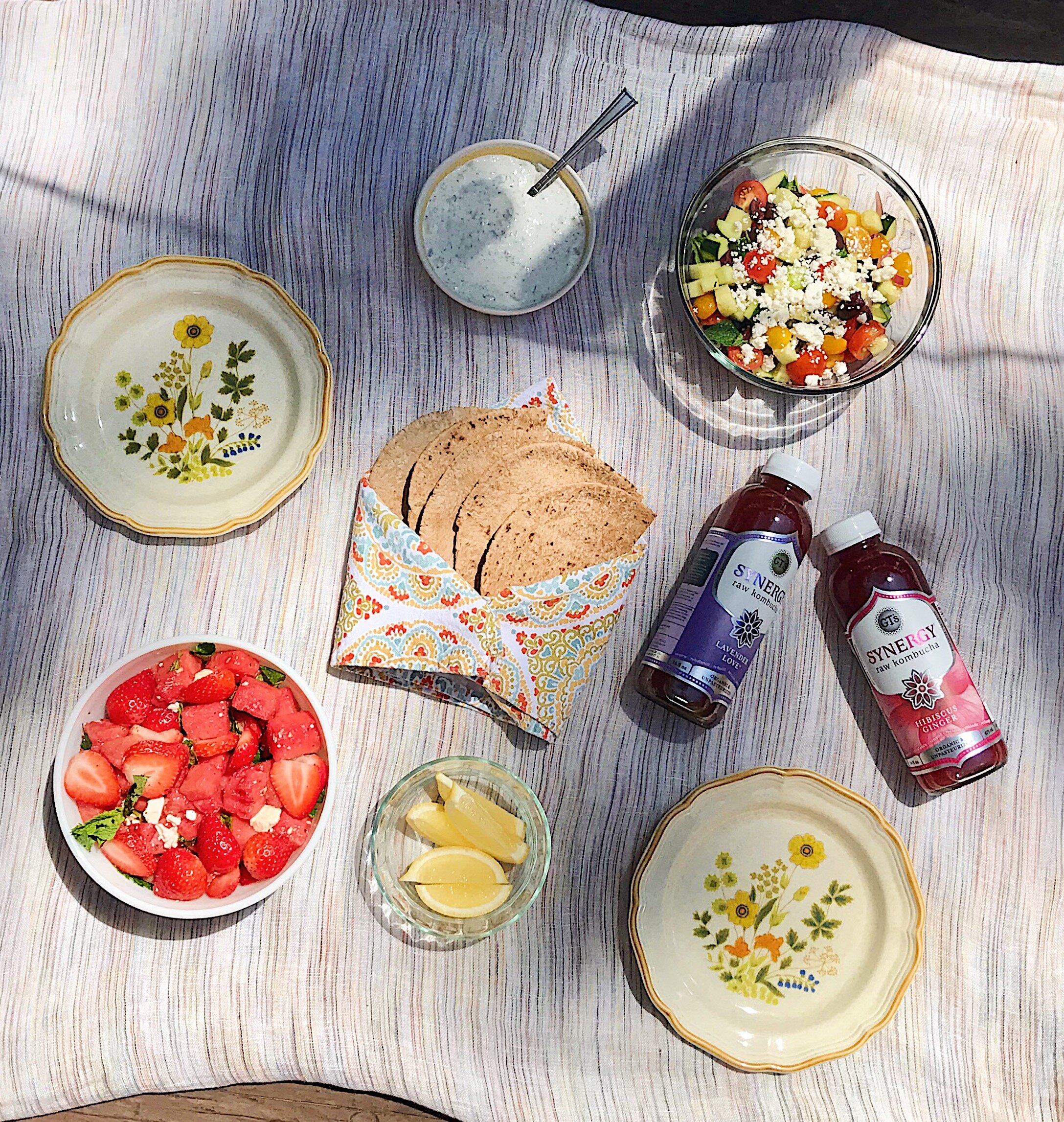This is a square, color photograph taken from above, showcasing a beautifully arranged picnic spread on a faint gray and white striped blanket. Central to the display is a colorful napkin holding a few slices of bread, surrounded by various delectable treats. To the right of the bread, there is a glass bowl containing lemon slices, and a bowl with a white yogurt dipping sauce with a spoon in it. Just left of this is a white bowl filled with a vibrant salad of strawberries, feta, and basil. Nearby sits a glass bowl of a refreshing cucumber, tomato, and feta salad. 

Accompanying these items are two decorative, cream-colored glass plates with floral designs—one located in the top left corner and the other in the bottom right corner of the image. Adjacent to the center, partially hidden below the blanket's stripes, are two bottles of Synergy Raw Kombucha. One bottle is labeled "Lavender Love" and the other "Hibiscus Ginger." Both feature white caps and colored labels purple and red, embracing the aesthetic harmony of the scene. The careful arrangement and variety of items exude a sense of casual elegance and inviting simplicity in an outdoor setting.